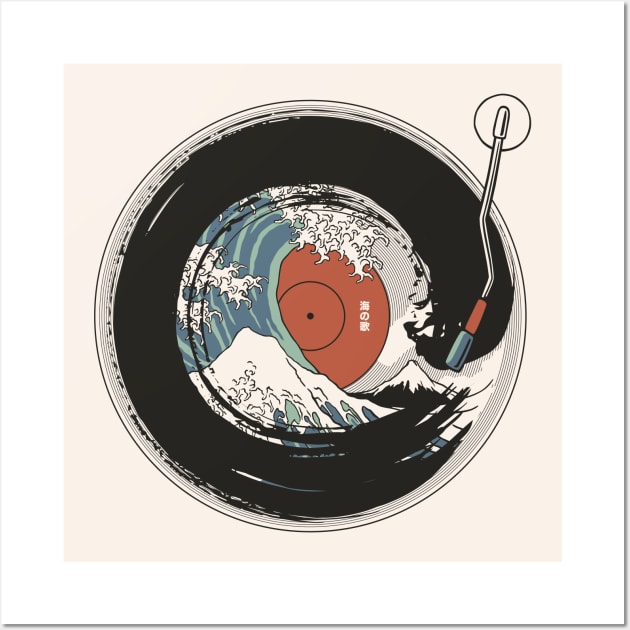This detailed drawing or painting features an LP record set against a cream-colored background, framed by a white border. The record itself is predominantly black along the edges but features intricate designs at its center. There, one can see a crashing wave rendered in dark blue-green and light mint green hues. Two mountains are depicted beneath the wave: the one on the left is green with a white peak, and the one on the right is black with a white peak.

The record's center is a burnt orange color, enhancing the contrast against the surrounding black. Above the record, a stylized record player needle and arm descend towards the disc, adding a tactile sense of motion and sound. Below the needle near the bottom left, there's a small red segment transitioning into a light blue piece, adding an additional splash of color.